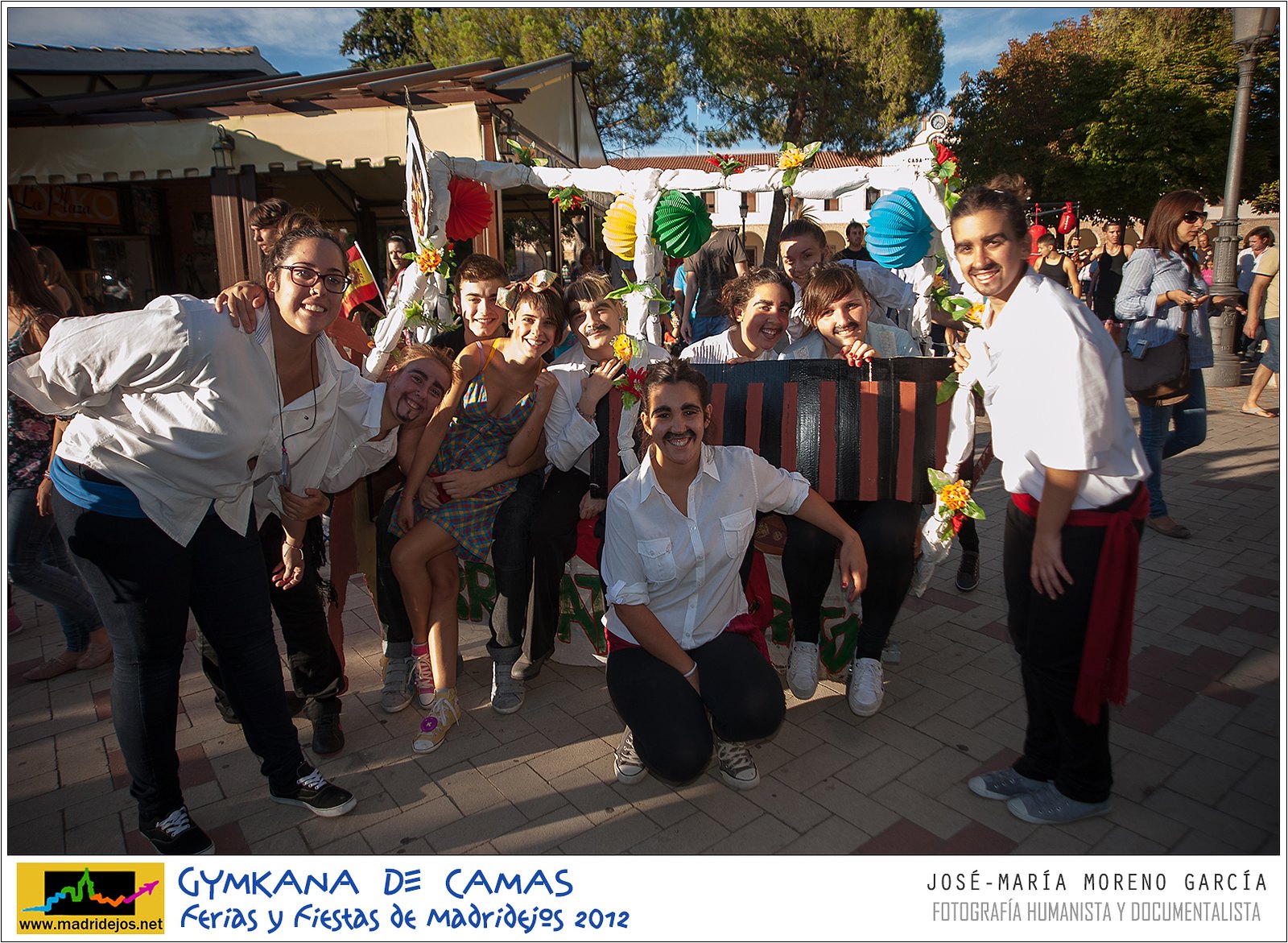The image captures a lively outdoor festival with numerous individuals participating, primarily dressed in white tops and black pants, complemented by either red or blue sashes around their waists. The festive atmosphere is palpable, with bright party decorations visible in the background, including vibrant colors like red, yellow, green, blue, and white. Predominantly, the people in the image are facing the camera, all smiling and exuding joy. Notably, some young ladies have painted facial hair such as goatees and mustaches, adding to the whimsical nature of the event.

The setting is an open, tiled area that resembles a large sidewalk or park, flanked by trees and a tan-hued, home-like structure to the left side of the image. A makeshift structure can be seen in the center. There are people in the background, engaged in their day-to-day activities, seemingly unfazed by the festivities, which adds a layer of everyday life to the scene. To the right, there's a black streetlamp and more people walking. The ground is tiled and clearly defines the outdoor space.

In the foreground, besides two prominently featured girls in coordinated outfits with white button-down shirts, black pants, and red sashes, there is a woman slightly off-center to the left, sitting and smiling. The details at the bottom of the image include a logo of a city skyline with a plane, and Spanish text crediting the photograph to Jose Maria Moreno Garcia, suggesting a possible Hispanic or specifically Spanish cultural celebration. Additionally, there’s a website address, www.madriddejos.net, further hinting at a connection to Madrid.